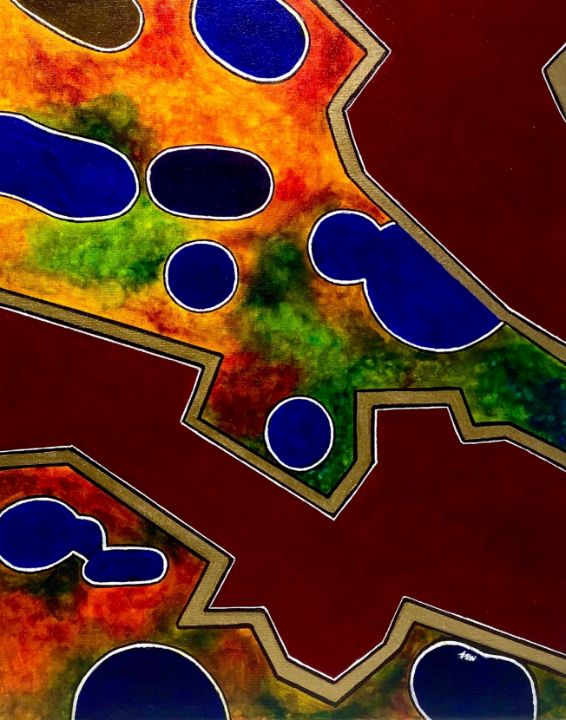The image is an abstract painting featuring a complex interplay of jagged shapes, vibrant colors, and distinct textures. Dominating the composition are two large, irregularly jagged brown shapes, one originating from the upper right-hand corner, bordered by striking gold lines. These jagged brown areas create a dynamic contrast against a background filled with smudged and modeled hues of red, green, and yellow, reminiscent of stained glass. Interspersed among these vivid colors are solid dark maroon sections, adding depth and intensity.

Centrally located within the vibrant background are blue circular blobs, each surrounded by a thin white border that gives them a cell-like appearance. These blobs are superimposed on the fuzzy, bright sections, where hues of green, orange, and red blend together seamlessly. Additional dark blue and black shapes, similarly outlined in white, scattered across the image, enhancing the painting's intricate and abstract nature.

From the upper to lower sections, the painting reveals a repeated pattern of brown jagged pieces with gold edges, contrasted against a colorful backdrop, dotted with blue blobs and segmented by solid dark sections. This repetition and the bold, contrasting elements create a visually striking and richly detailed abstract work.